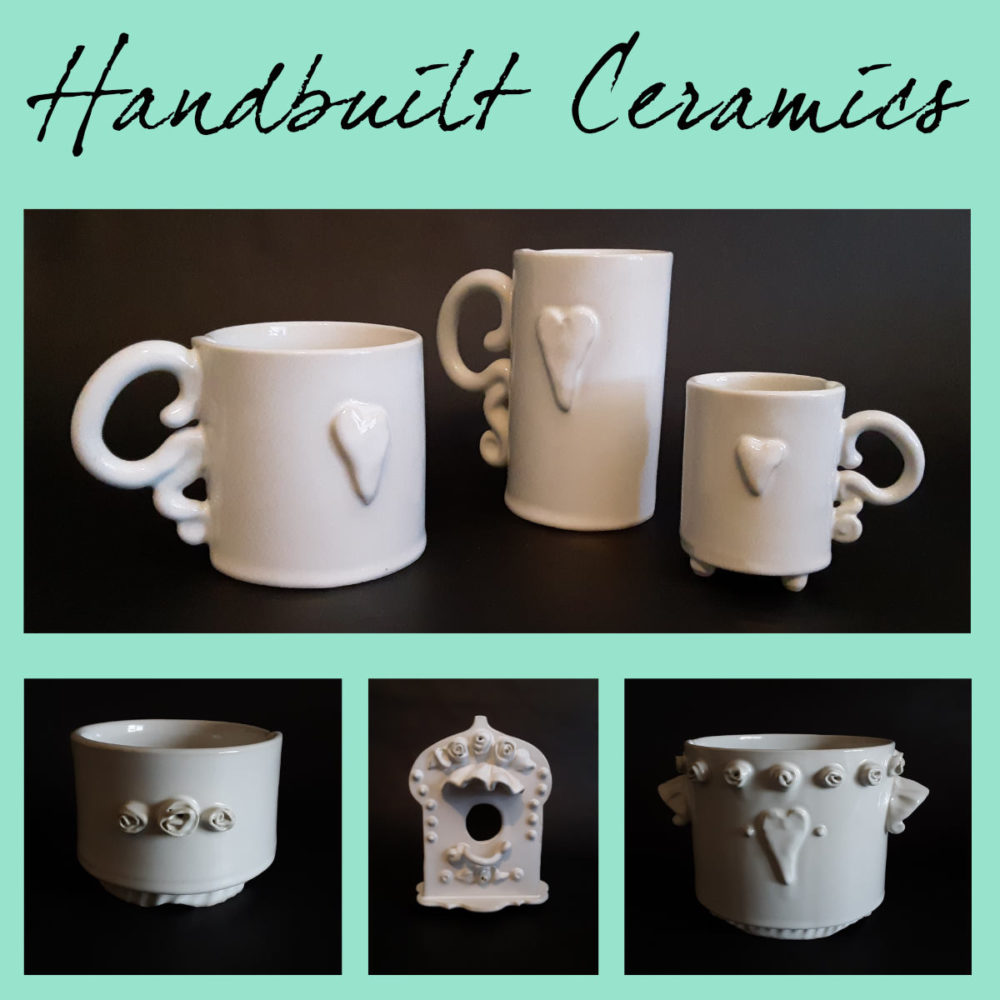The image features an advertisement for handmade white ceramic cups against a mint green background. At the top of the image, bordered text reads "hand-built ceramics" in green. The advertisement includes four photos. The largest photo at the top displays three distinct ceramic mugs: a tall one resembling a beer mug and two smaller ones akin to coffee mugs, each adorned with protruding rustic hearts and elaborate swirly handles. Below this main photo are three smaller images: the first shows a small bowl decorated with roses, the second might depict a birdhouse, and the last presents another bowl featuring roses, a heart, and small handles. All items showcased are monochromatic white, enhancing their handcrafted appeal.